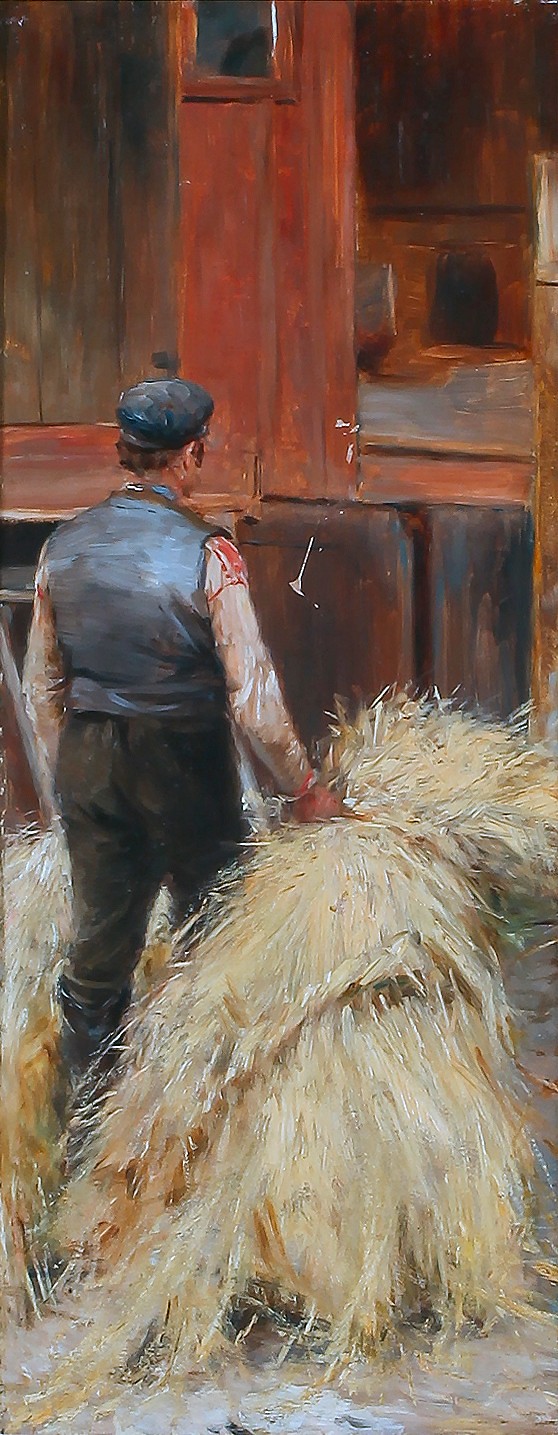The painting depicts a man viewed from behind, positioned on the left side of the composition. He faces a wooden building, presumably a barn, characterized by its dark brown lower wooden structure and partially visible red upper section with an open door revealing an interior space with a wooden fireplace. The man wears a gray newsboy cap, a gray vest over a white shirt, and black pants, possibly with working boots. His right hand is extended towards a large pile of light yellowish-tan hay. The ground beneath him is a light tan color, possibly snow-dusted. The setting conveys a rustic, agricultural environment.